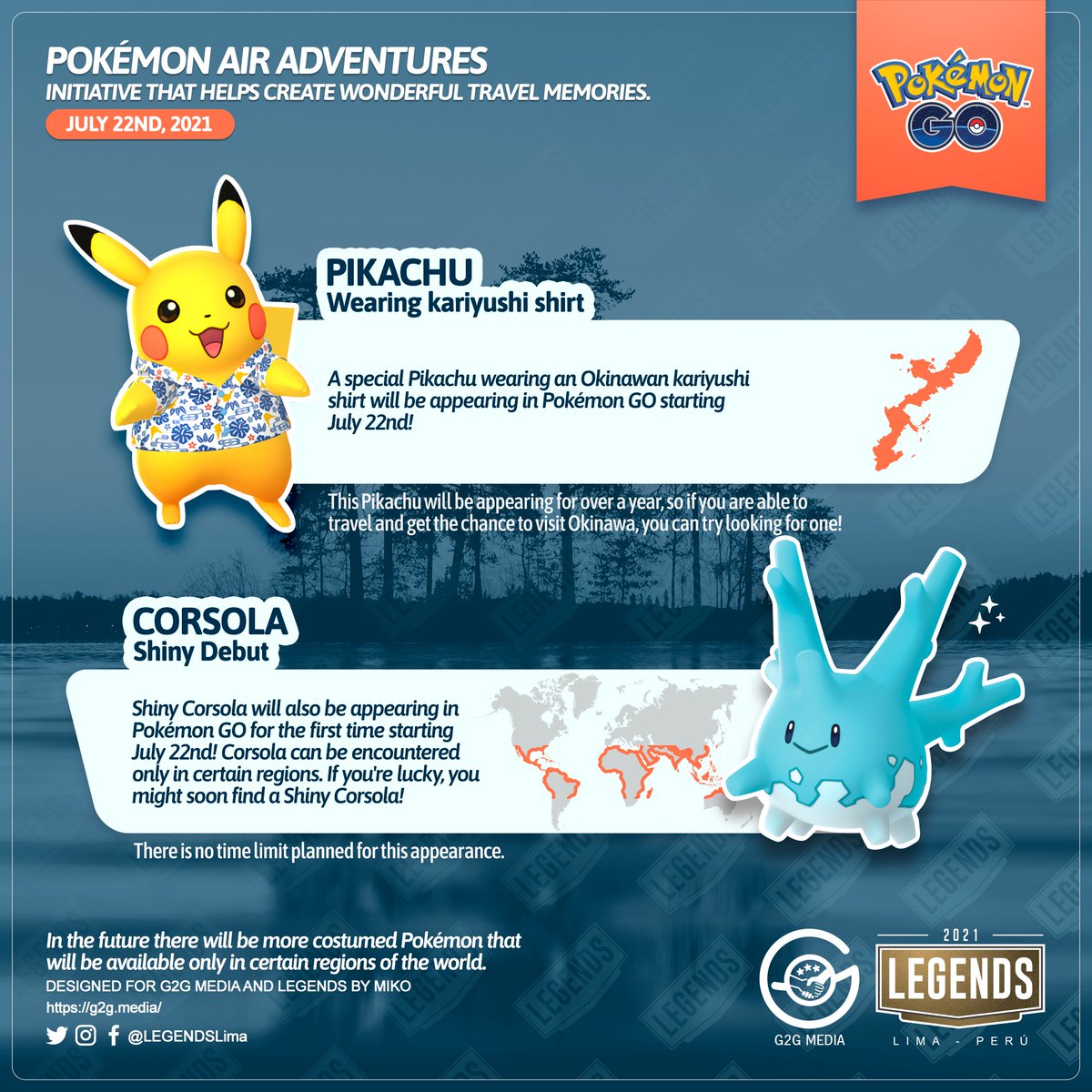**Screenshot from Pokémon Go Website Advertising "Pokémon Air Adventures"**

In this vibrant advertisement from the Pokémon Go website, a dynamic blue background featuring blue trees sets the stage. The text "LEGENDS" is prominently displayed across the screen in a transparent, white-outlined, and black lettering format.

Key elements of the promotion include:

- **"Pokémon Air Adventures" Initiative**: Highlighted in white text, this initiative is designed to help create memorable travel experiences.
- **Date**: July 22nd, 2021, marked with white text inside an orange circle.
- **Logo**: The Pokémon logo is positioned in the upper right-hand corner on a small banner.
  
A prominent feature of the advertisement includes an image of Pikachu, the iconic yellow Pokémon with red cheeks, donning an Okinawa Kaiyushi shirt. Accompanied by the text "Pikachu wearing a Kaiyushi shirt," the ad announces the special appearance of this Pikachu in Pokémon Go starting July 22nd. This special Pikachu will be available for over a year, offering players a chance to find it while traveling, especially to Okinawa.

Additionally, the ad highlights the debut of Shiny Corsola – a coral-like Pokémon. Shiny Corsola, distinguishable by its blue coral reef appearance, will also be appearing in Pokémon Go for the first time starting July 22nd. Although Corsola can only be encountered in specific regions, lucky players may find a Shiny Corsola.

The advertisement also teases the future introduction of more costume Pokémon, available exclusively in certain world regions.

Designed by Miko for G2G Media and Legends, the ad includes social media handles for Twitter, Instagram, Facebook, and contact information for Legends Lima. At the far bottom right, G2G Media and the year 2021 along with Legends Lima, Peru are noted.

Overall, this advertisement serves as a vibrant and inviting call to Pokémon Go players, encouraging exploration and a special in-game experience.